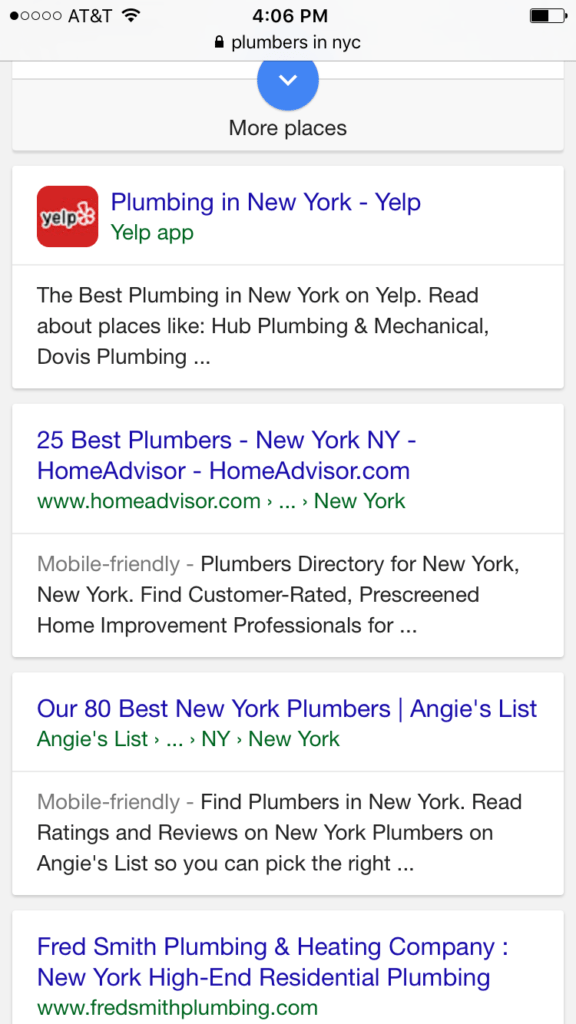In the screenshot set against a light gray background, various informational elements are displayed on a smartphone screen. The upper left corner indicates the reception status with one out of five bars, accompanied by the text "AT&T" in black. The Wi-Fi icon is also visible, signifying an active connection. Centered at the top is the time, reading 4:06 p.m. Below the time, large bold text reads "Plumbers in New York City."

In the upper right corner, the battery icon shows a half-charged status. Below the main title, within a white box, the Yelp icon appears as a red box with black letters reading "Yelp." Next to the icon, the text "Plumbing in New York" is displayed in blue. Beneath the Yelp section, green text states, "The best plumbing in New York on Yelp," and mentions notable plumbing services such as Hub Plumbing and Mechanical, and Davis Plumbing. 

The following section exhibits blue text titled "25 best plumbers New York New York HomeAdvisor HomeAdvisor.com." Below this, in green, the URL "www.HomeAdvisor.com New York" is shown, emphasizing the mobile-friendly nature. The description continues, concluding with a service promise: "Find customer-rated, pre-screened home improvement professionals."